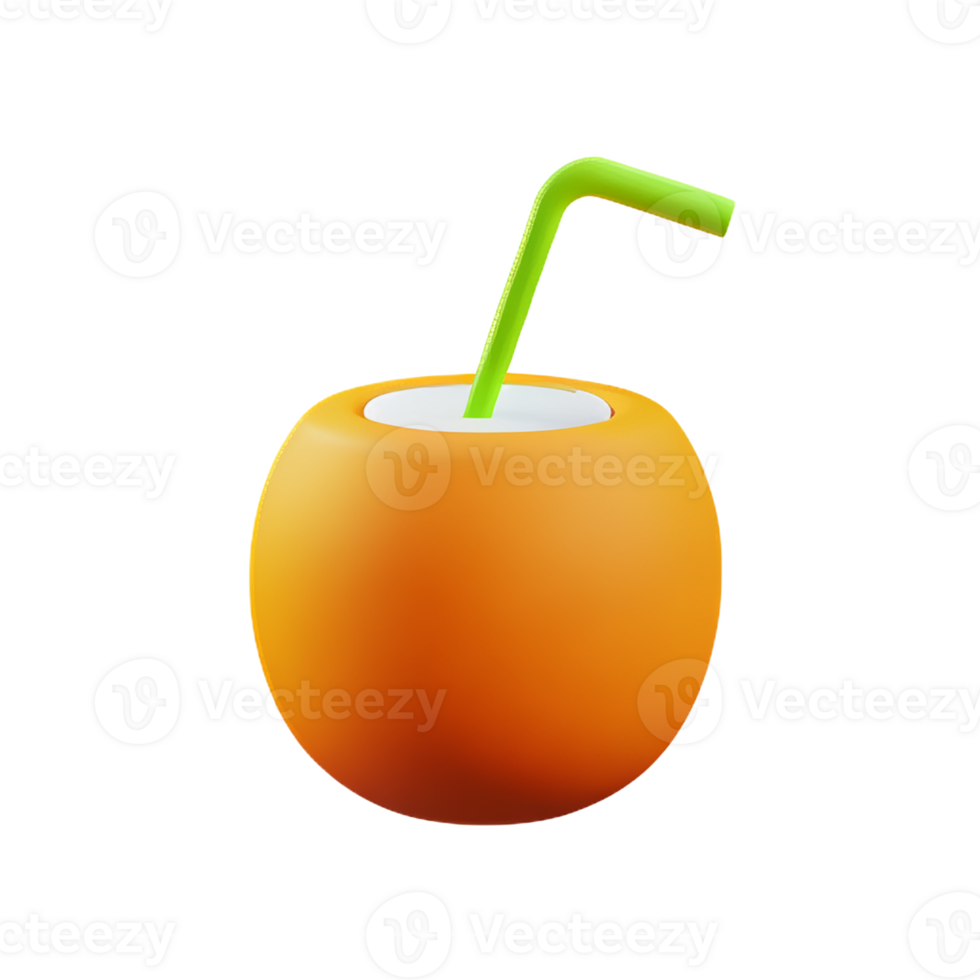The image depicts a product photograph of a child’s cup designed to resemble an orange. The cup is predominantly orange, featuring a white lid that is slightly smaller in diameter than the cup itself. A green straw protrudes from the lid, bent at a 90-degree angle and tilted slightly off-center. The background is pure white, emphasizing the cup’s vibrant colors. Throughout the image, there is a recurring watermark that spells "Vecteezy" alongside a logo consisting of a white circle containing a cursive 'V' with a curl at the end. The cup appears to be made of plastic and likely holds around 10 ounces of liquid. Its playful, fruit-like design suggests it is intended to appeal to children.